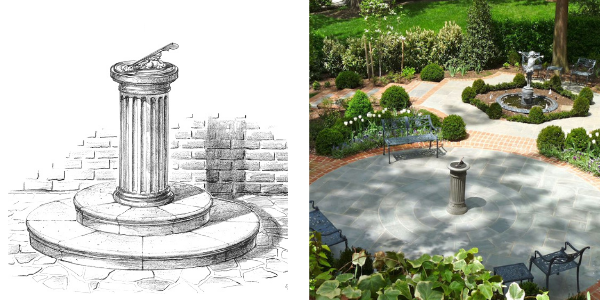The image showcases two side-by-side depictions of a sundial: the left one is a black-and-white drawing, while the right one is a color photograph. In the drawing, the sundial sits atop a light gray circular base, mounted on a column with vertical etchings. This column stands on two stacked circular platforms, with the larger one at the bottom. The background includes a brick wall casting a darker shadow on the light gray setting. 

The photograph on the right captures the sundial from a top-down perspective, highlighting its dark gray hue and the lighter yellow ring encircling its top. This sundial is similarly placed on a gray column that extends downward to a light gray concrete surface. Situated in a park, the scene includes a dark gray bench to the upper left and green plants in the vicinity. There is a statue atop a water fountain in the far background, surrounded by green bushes and shrubs with some white flowers. The area is dappled with sunlight and shade, with stone pavers providing a flat surface, complemented by black metal chairs at the bottom corners. This comparison highlights both the artistic interpretation and the real-world setting of the sundial, set within a well-manicured garden environment.